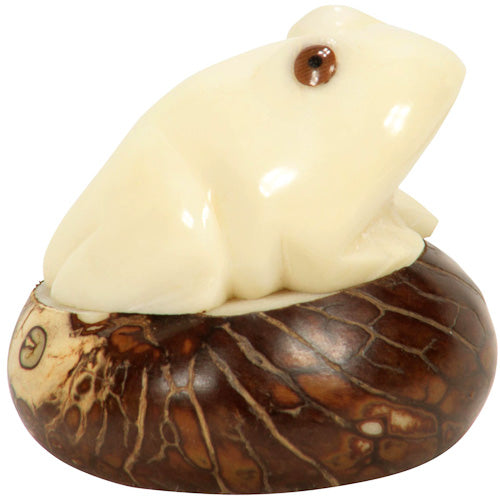This photograph depicts a finely carved figurine of a frog, crafted with intricate details and remarkable texture. The frog itself is an off-white hue with subtle yellowish tones and features expressive brown eyes with black pupils. It is perched on a small, polished pedestal. This pedestal, shaped like a doughnut or rounded oval, exhibits a striking pattern with brown and white veins, adding to its aesthetic appeal. The smooth, gleaming surface of the pedestal suggests it could be made from either a distinctive type of wood or a polished stone or marble, though its exact material remains uncertain. The craftsmanship is of high quality, emphasizing the texture and gleam of both the frog and the pedestal, creating an overall visually appealing art piece.